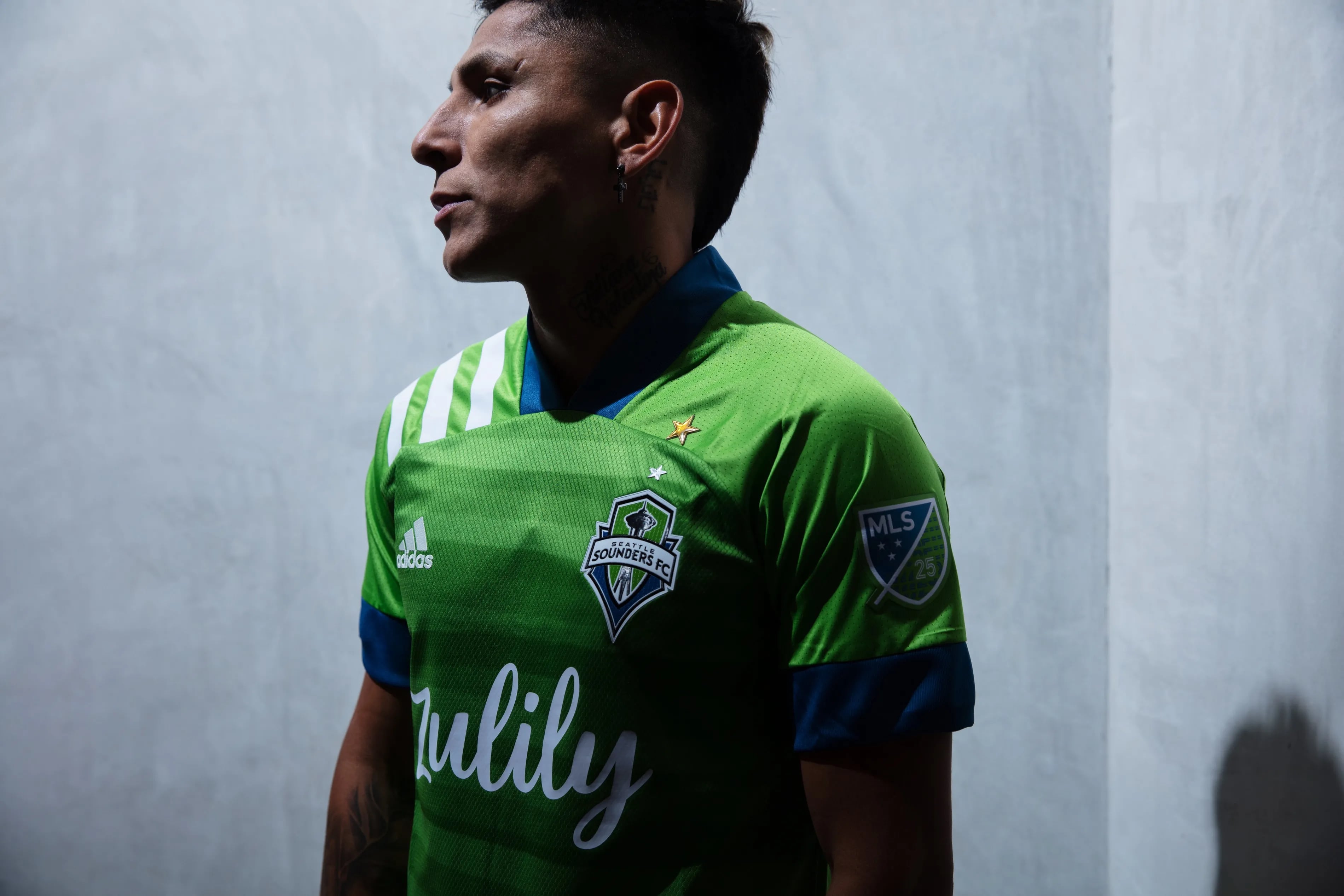The image depicts a soccer player from the MLS, specifically from the Seattle Sounders FC. He appears to be Hispanic, in his 20s or 30s, with short, dark hair. The player is positioned at the center of the image, looking towards the right. He is wearing a predominantly green jersey with blue accents. The jersey prominently features the "Zulily" logo in white cursive on the chest. On the player's right shoulder, there is an MLS patch, followed by another unreadable patch with a gold star above it. The left shoulder showcases white stripes with the Adidas symbol beneath them. The background consists of empty grayish-white walls, with a small shadow on the right side, suggesting a simple indoor setting. This detailed composition and the attire clearly identify him as an MLS player.